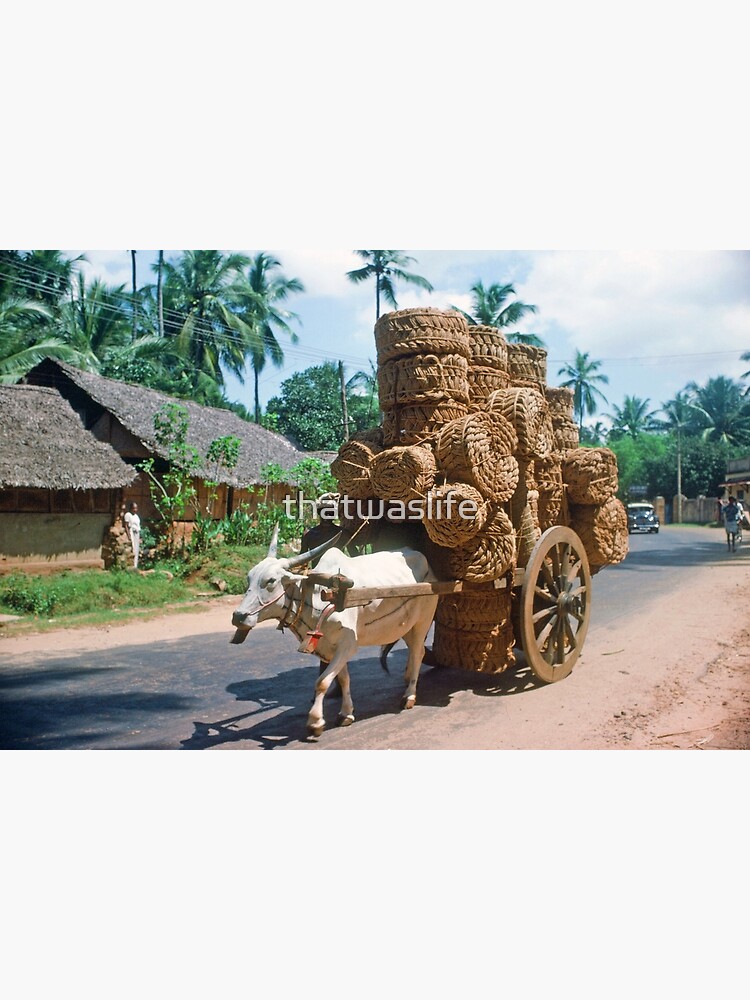A vivid color photograph captures a serene scene likely set outside North America. Dominating the image is a robust white oxen with long, curved horns and a black beard, pulling an overloaded wooden cart. The cart is filled to capacity with various woven materials, including rags, fabrics, and circular bundles, all tied with ropes. This simplistic yet sturdy cart moves along a paved road bordered by expansive areas of dry dirt. Surrounding this path are numerous huts constructed with thatched roofs, indicative of natural, local materials. In the background, lush palm trees sway gently, and a vintage automobile approaches, adding a touch of contrast to the rural setting. Overlaid on the image is the poignant text, "That was life," encapsulating the scene's nostalgic and timeless essence.